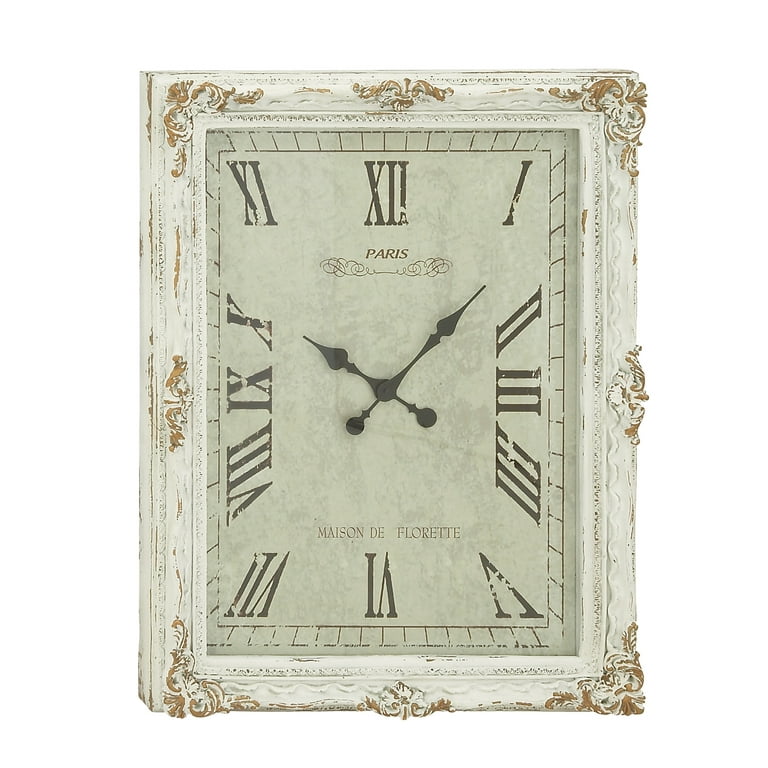This image depicts a vintage shabby chic rectangular clock featuring a distressed white wooden frame with intricate floral and cursive swirl patterns, giving it an antique appearance. The frame, painted white and sanded to achieve a worn, shabby chic look, shows some tan-colored spots where the paint has been rubbed off. The clock face, designed in a worn mottled gray, displays Roman numerals in dark gray. The face indicates the time as approximately 10:07 with its similarly aged, dark gray hands. Underneath the Roman numeral XII, the face reads "Paris," followed by the elegant script "Maison de Fleurette" above the Roman numeral VI, reflecting its French charm and vintage aesthetics.